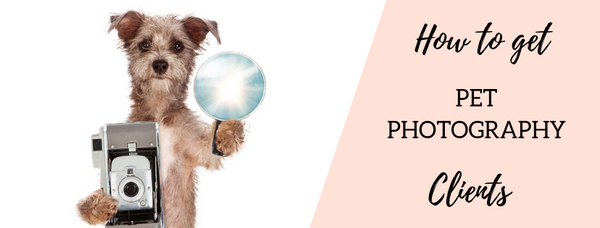The image is a detailed advertisement for pet photography services. It features a photorealistic small brown terrier with short, shaggy fur and a patch of white on its chest. The dog is standing upright and is positioned against a plain white background with no borders on the left side of the image. The terrier directly faces the camera, holding a vintage black and white camera in one paw and a flashbulb in the other. The dog has floppy ears, dark brown eyes, and a brown nose.

To the right of the dog, the background transitions into an orangish-cream parallelogram shape. This section of the image contains black text, with a headline written in cursive that reads, "how to get," followed by "PET PHOTOGRAPHY" in large print, and "clients" underneath in cursive. The juxtaposition of the white and colored backgrounds and the clear promotional intent make this image a compelling advertisement capturing the essence of pet photography services.